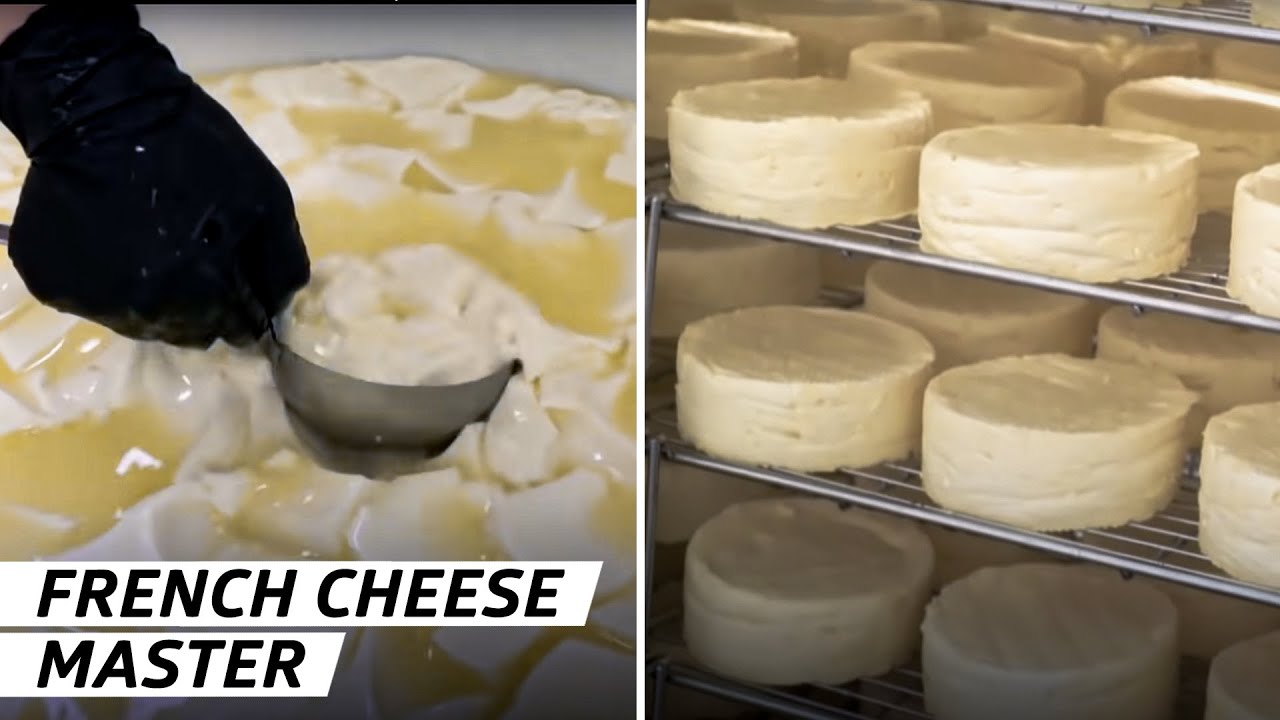The image is a two-panel photograph showcasing the meticulous process of cheese making by a French cheese master. In the left panel, a gloved black hand is seen using a metal ladle to scoop a gooey, ooey mixture of white and yellow cheese from a vat, emphasizing the intricate craft involved in cheesemaking. Written in black letters on a white background is the label "French Cheese Master," indicating the expertise of the individual. The right panel features metal racks filled with cylindrical cheese rounds, arranged in rows, resembling layer cakes or small hockey pucks. These cheese rounds are set on three visible shelves, each lined with multiple rows of neatly placed, drying cheese, highlighting the cheese's progression from creation to preservation.